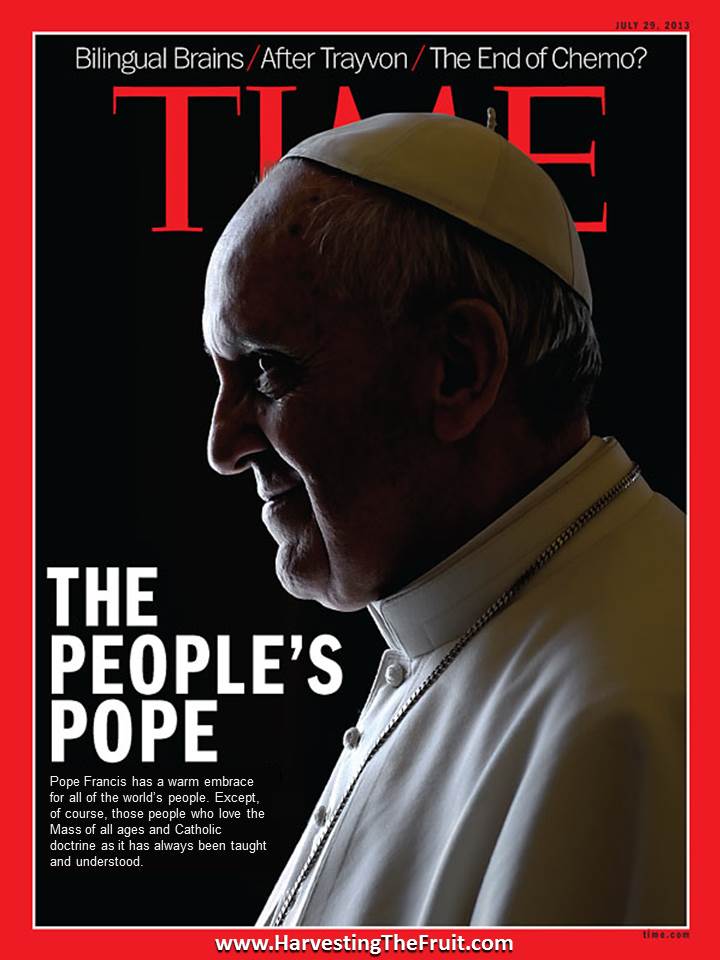This vertical, rectangular cover of Time Magazine prominently features a side profile of Pope Francis, facing left. His head, partially obscuring the large, red "TIME" masthead, is crowned with a white zucchetto, while he wears his traditional white papal robe and a long, silver chain around his neck. The photograph captures a slightly shadowed, yet warmly smiling Pope against a solid black background, bordered by a striking red frame.

Above the "TIME" logo, in white text, are the headlines: "Bilingual Brains / After Trayvon / The End of Chemo?" On the lower left-hand side of the cover, bold white capital letters declare him as "The People's Pope." Below this, a small paragraph reads: "Pope Francis has a warm embrace for all of the world's people—except, of course, those who love the mass of all ages and Catholic doctrine as it has always been taught and understood."

Finally, at the bottom, a small detail directs readers to "www.harvestingthefruit.com."